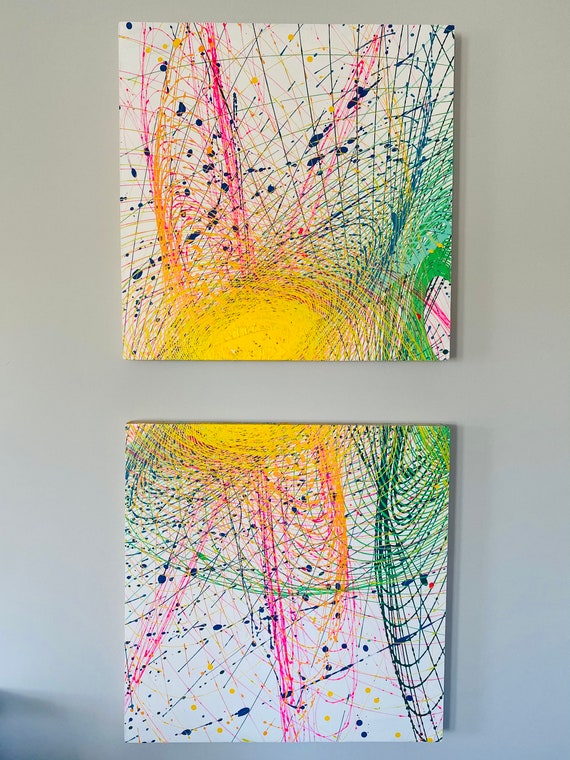This image features a pair of vibrant, modern art pieces displayed on a gray wall. The two square canvases, each with a white background, are hung one above the other with a small gap in between. The artwork on both canvases is characterized by a profusion of colorful swirls, splatters, and lines, predominantly in shades of pink, green, blue, and black. Central to the composition is a large yellow circle, split horizontally across the two canvases: the top half resides at the bottom of the upper canvas, while the bottom half appears at the top of the lower canvas. Surrounding the yellow circle are green rings, interspersed with some orange, and accented by vertical pink lines. These elements align seamlessly, suggesting the canvases were once a single artwork, now divided to create a cohesive yet dynamic visual connection.